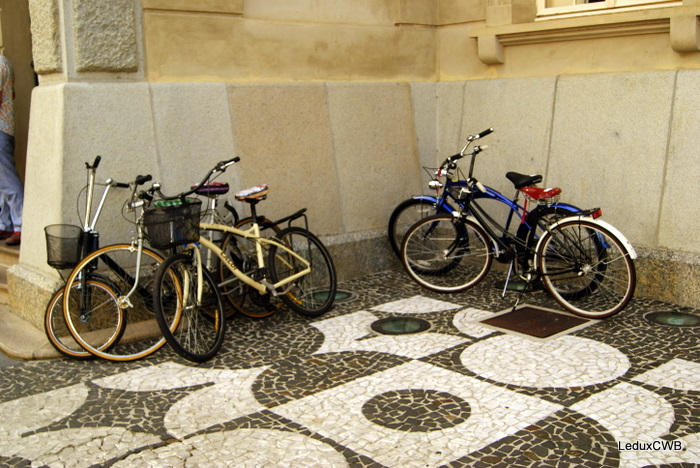In this detailed outdoor scene, five bicycles of various colors and types are stacked against the corner of a large, old stone building. The structure, which could be a church or a courthouse, has a prominent stone facade with stones about six feet tall. Above this is a window barely visible in the top right. One bicycle is white with a red seat and tall handlebars, while another is a kid's bike with a basket on the front, reminiscent of a Stingray bike. A typical men's bike with a basket is also present, along with a blue bicycle in the background. Three of the bikes lean against the wall, and two are supported standing. The ground is covered in modern tiles featuring a circles and squares pattern in gray and black, adding a contemporary touch to the historical setting.